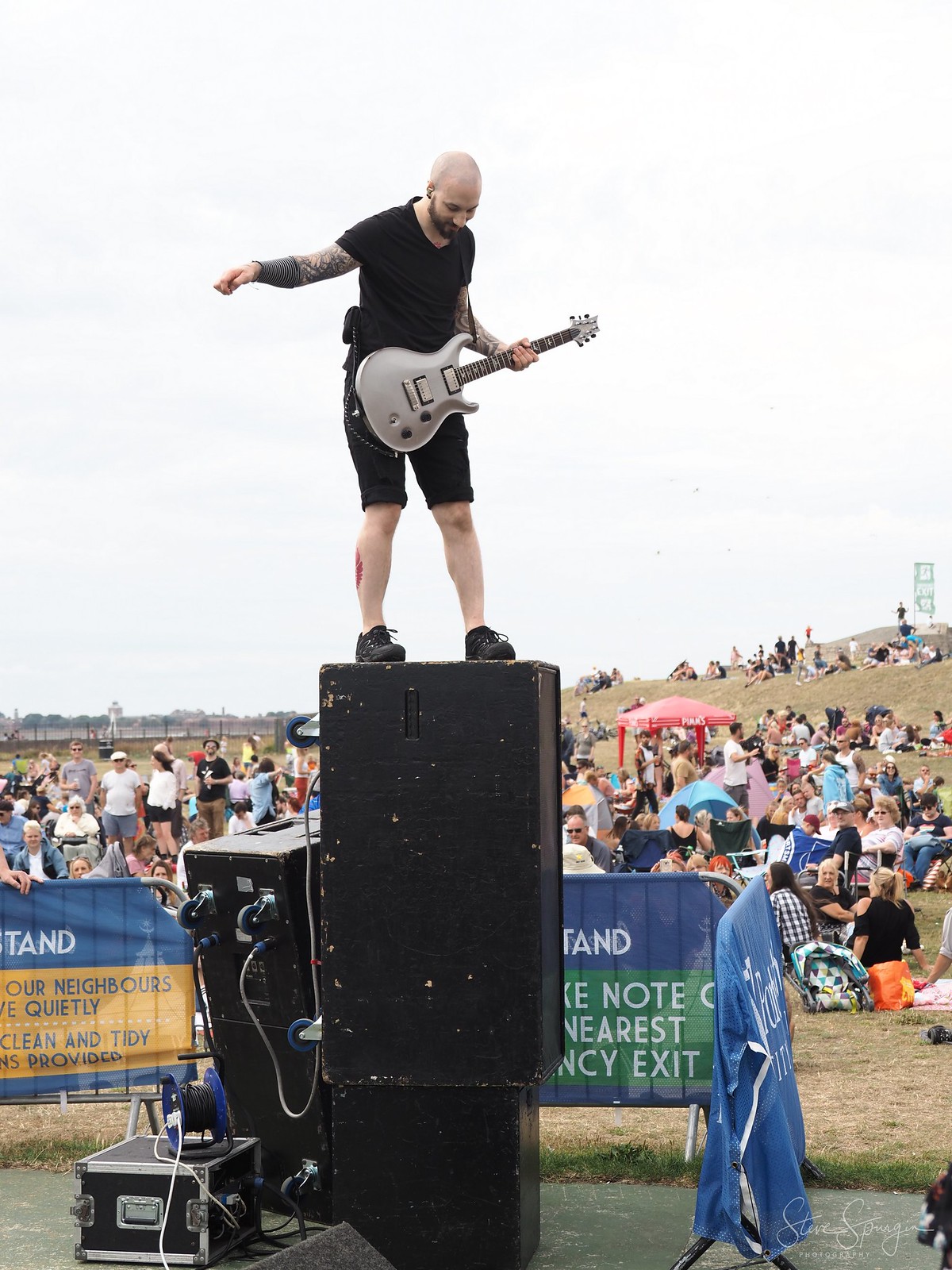In this detailed portrait-oriented color photograph, the focal point is a white, bald man with a scruffy brown beard, standing and playing a gray electric guitar atop a large black speaker at an outdoor concert event. He is dressed in a black t-shirt, black shorts, and black sneakers, and sports an extensive full sleeve of tattoos on his right arm. Behind him stretches a large grassy field with a gently sloping hill to the right, populated by concertgoers sitting and standing, dressed in various colors. About a kilometer away on the left, a building is visible. The sky, which occupies about half of the image, serves as the backdrop against which the man stands prominently. There are also blue signs with white lettering near the speakers, likely providing information related to the event. The atmosphere evokes the sense of a lively musical festival, with the man's central positioning on the speakers underscoring the vibrant energy of the scene.